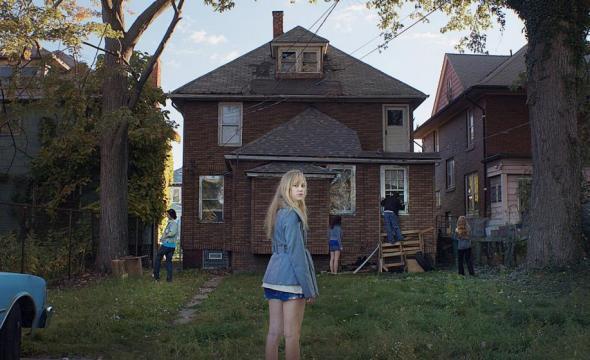The photo depicts a group of young people in the backyard of a brown brick house situated in a neighborhood. Centered in the image is a young blonde woman in a blue jacket that covers her shorts and shirt. She stands with her back to the camera, but her face is turned towards it, revealing her expression. The house itself is detailed with white-framed windows and a large expanse of greenery in front, indicating it is the backyard. 

To the left of the house stands a young man with dark hair, dressed in a blue jacket and blue jeans. Another young woman with dark hair, wearing a blue shirt and blue shorts, is positioned to the right of the central blonde girl. Further to the right, a young person in a blue jacket and jeans is on top of a wooden structure, peering into one of the house’s windows. Another young girl in a blue jacket with dark pants stands even further to the right. 

The background features two more brownish-colored houses, one partially obscured by a large tree with lush green leaves on the left. A thick tree is also visible on the right edge of the image. The sky above is bright blue with light white clouds, suggesting a clear day. There are additional items in the scene, including a camera on a tripod and what appears to be an older blue car with its front part visible on the left side of the photo. Textural elements, such as a tire and possibly some construction activity or renovation work around the houses, add to the scene’s detailed, busy environment.